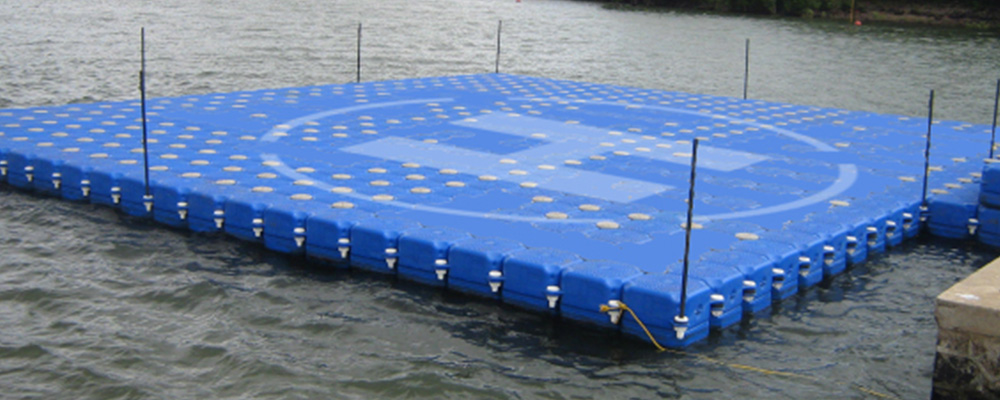The photograph captures a floating helipad situated on murky gray water, designed to be a portable landing pad for helicopters. The helipad is constructed from interlocking blue blocks of buoyant material, resembling bricks or heavy plastic, which feature round holes on the surface likely contributing to its buoyancy. The most prominent feature is a large, light blue "H" encircled in the middle, marking it as a landing site. Surrounding the helipad are white poles or spikes, possibly for stability or to tether the structure with ropes, as evidenced by a yellow rope attached on the bottom left corner. Access to the helipad is provided by a set of blue stairs at the right, leading up to a stone-edged pier visible in the bottom right corner of the image. The bright blue color of the helipad contrasts starkly with the muddy water, making it easily identifiable from the air.